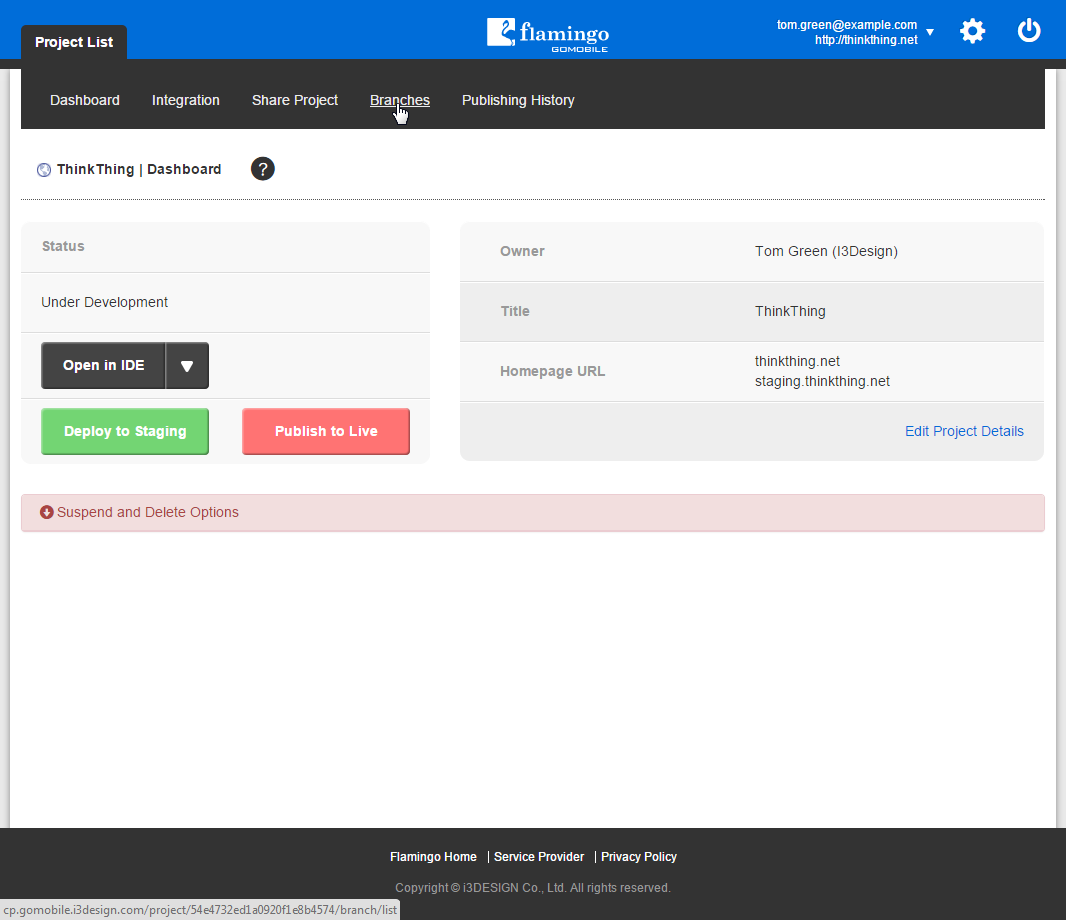This is a screenshot of a software interface. At the top, there is a horizontal blue bar featuring a centered logo: a white square with a blue flamingo inside it, next to the word "flamingo" in lowercase white letters. To the right of the logo, contact details such as an email address and website are displayed, accompanied by a drop-down arrow, a settings icon, and a power icon.

On the left side of the interface, there's a vertical blue rectangle, outlined in black, containing a list of navigation options in white text. At the top, it reads "project list." Below this heading, there's a horizontal black rectangle with "dashboard" in white text to the right of "integration," followed by "share project," and "branches," which is underlined and highlighted with a white hand pointer. "Publish history" is listed at the bottom of this navigation menu.

Below the navigation area, the background transitions to white. About three lines down, a blue circle is visible with the text "think thing" in gray to the right of it. A vertical gray line separates the dashboard from a black circle containing a gray question mark.

Further down, the interface displays the status "under development," alongside several buttons: an "open in IDE" button with a drop-down arrow, a green "deploy to staging" button in white text, and a red "publish to live" button, also in white text. To the right of these buttons, there is a gray rectangle providing information about the owner, title, and home page URL.

At the bottom of the interface, a light pink horizontal rectangle spans the entire width of the page. Inside this rectangle, there is a circle with a white element inside it, and to the right, text that reads "suspend and delete options."